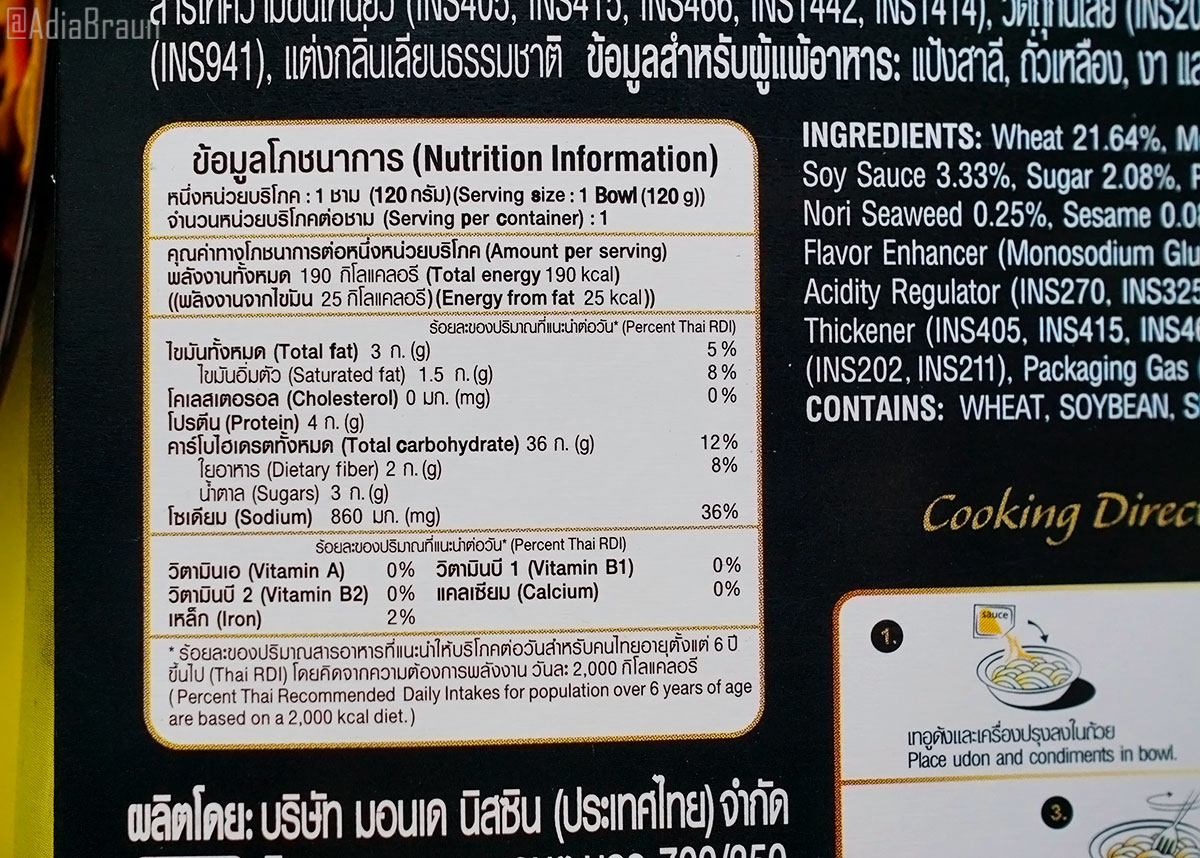In this image, we see the back of a product label, predominantly black with white print. In the upper left corner, a light watermark displays the name "Adia Braun." The text is primarily in a foreign language, which makes understanding all the details challenging. However, to the right of the nutritional information, several ingredients are listed: wheat (21.64%), soy sauce (3.33%), sugar (2.08%), flavor enhancer (monosodium glutamate), acidity regulator, thickener, and packaging gases. Additionally, there's a critical note stating, "Contains wheat, soybeans." In the lower right corner, an illustration provides directions—it seems to involve adding a packet of sauce to cooked pasta or noodles. This visual guide suggests a serving suggestion for the product.